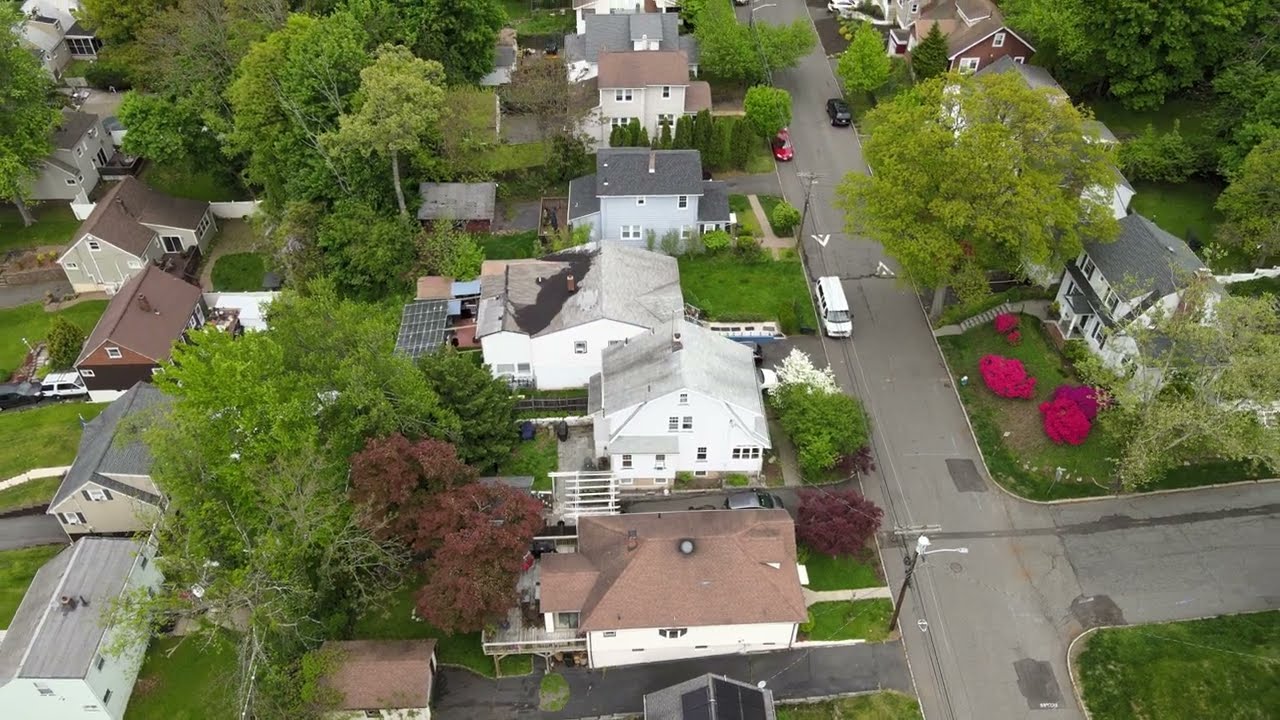The image is a high aerial photograph, likely taken by a drone, capturing a peaceful residential neighborhood during a bright, mostly sunny day in spring. The angle of the photo is three-quarters, revealing a detailed view of the area with six houses prominently lined up along a central block. Most of the houses are multi-story and exhibit a variety of styles, including ranch and Cape Cod. Their roofs come in different colors, such as red, light gray, dark gray, and brown, with one house even featuring solar panels in its backyard.

The houses are set amidst lush greenery with blooming trees scattered throughout the properties, showcasing the fresh, vibrant green of spring. Some yards have beautifully manicured pink and white flowering bushes, while each property seems to have well-maintained lawns, driveways, front yards, and backyards.

Two streets run vertically through the image, providing on-street parking where several vehicles, including a white van, a red car, and a black car, are parked. Additionally, there's a perpendicular street branching off to the lower right of the photo, just partially in view. This meticulously maintained, middle-class neighborhood exudes a serene and inviting atmosphere, enhanced by its organized layout and flourishing natural beauty.